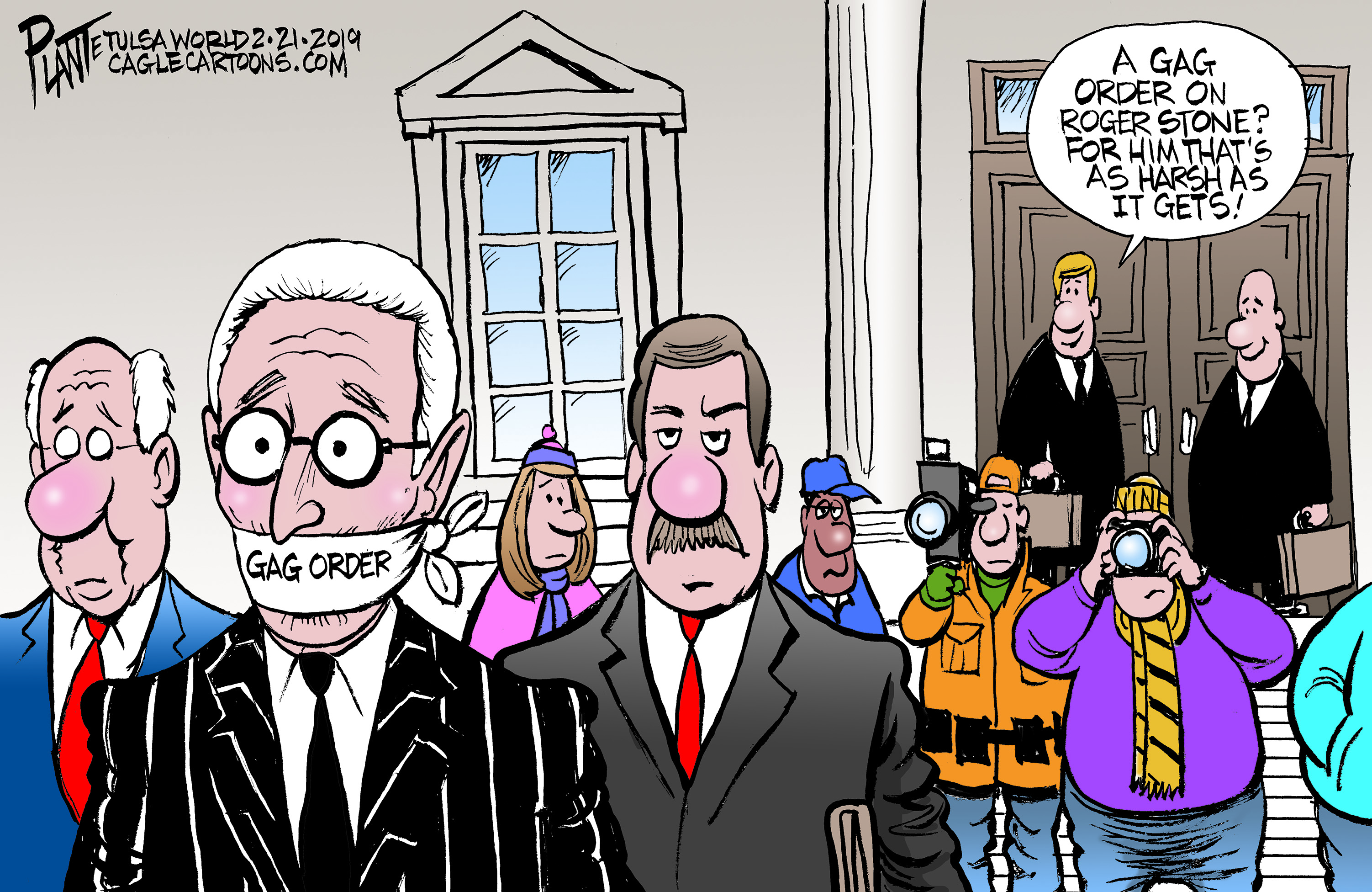This detailed cartoon by Bill Plant, featured in the Tulsa World on February 21, 2019, humorously depicts Roger Stone with a gag order. Stone, easily recognizable by his white hair, is shown wearing a black and white pinstripe suit, black tie, and white shirt, with a white bandana covering his mouth, labeled "gag order" in black letters. He stands in front of a courthouse, flanked by two individuals who appear to be his lawyers—one in a blue suit with a red tie, and the other in a dark gray suit, also with a red tie and a mustache. They seem to be holding onto Stone as paparazzi and media representatives crowd around, capturing the moment. The background includes various onlookers dressed in winter attire: a woman in a pink suit, a bystander in a blue hat and jacket, an individual in an orange jacket with a camera, and another person in a purple shirt with a yellow scarf, also taking pictures. Additionally, we see part of the turquoise jacket of a bystander at the edge of the frame. Above this scene, two individuals in black suits converse, with one judge remarking, "A gag order on Roger Stone? For him, that's as harsh as it gets."